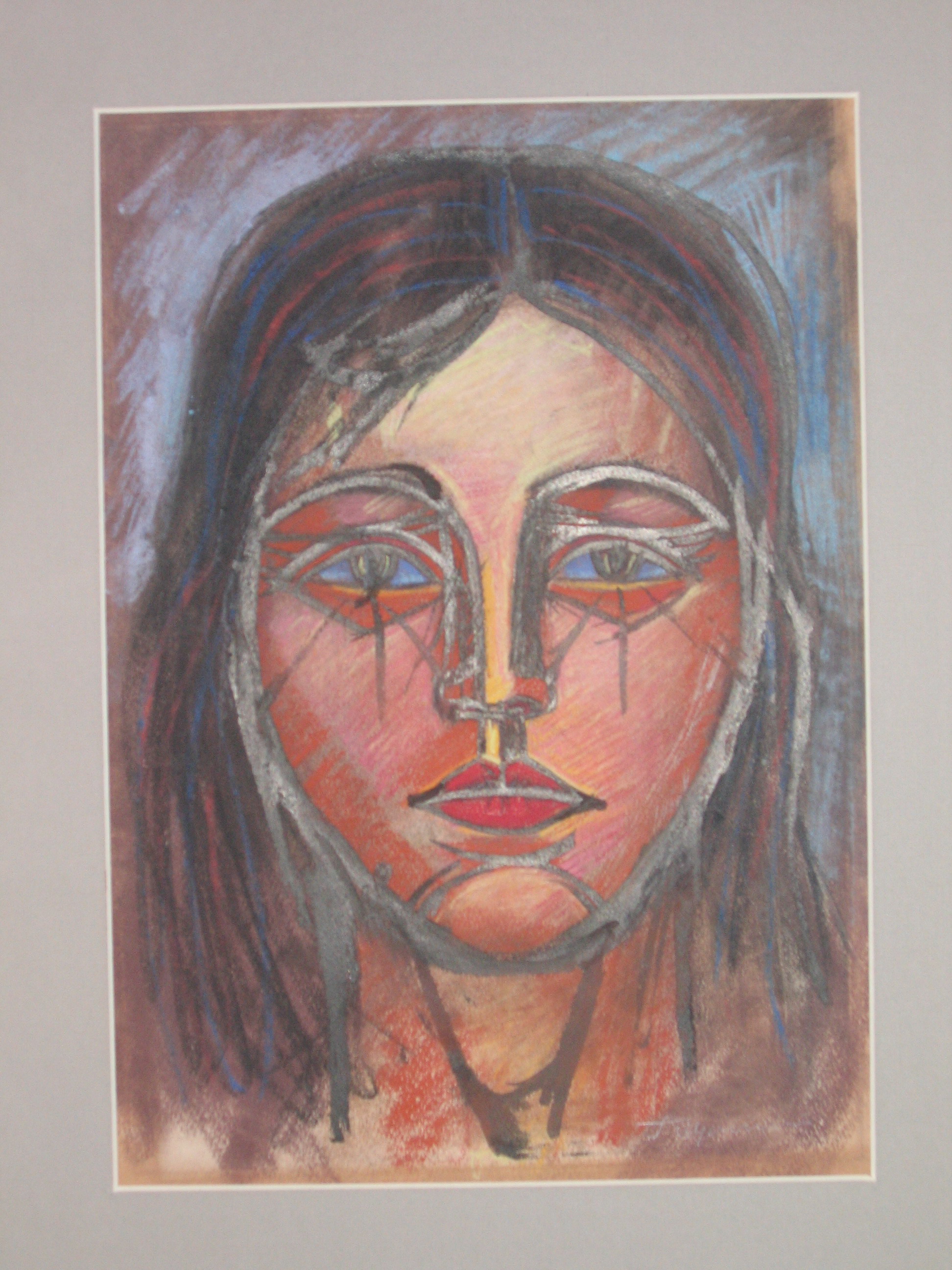This is a surrealist painting of a young girl's face, depicted with an expressionless yet solemn demeanor that conveys a sense of introspection. The girl, with shoulder-length brown hair interspersed with blue and red streaks, has striking green eyes accented by blue-tinged whites. Her complexion features various shades of tan and brown with white highlights, particularly on her forehead. She has cherry red lips, and her eyebrows are dark with light highlights beneath them, suggesting a detailed, thoughtful rendering of her features. Notably, there are three black lines descending from each of her eyes, adding to her melancholic appearance.

The painting employs a palette of black, white, gray, blue, red, tan, pink, and various shades of brown. The background consists of impressionist streaks of light blue, brown, and other colors, enhancing the surreal quality of the piece. The face and some portions of her hair on the right side are outlined in white, contributing to the artistic depth. The entire image is framed by a gray border, beyond which lies a white outline, confining the artwork within a distinct boundary. The medium used for the artwork could be paint or colored pencils, creating a texture that is hard to definitively pinpoint. There is no text or signature on the painting, focusing the viewer's attention entirely on the haunting, contemplative face of the girl.